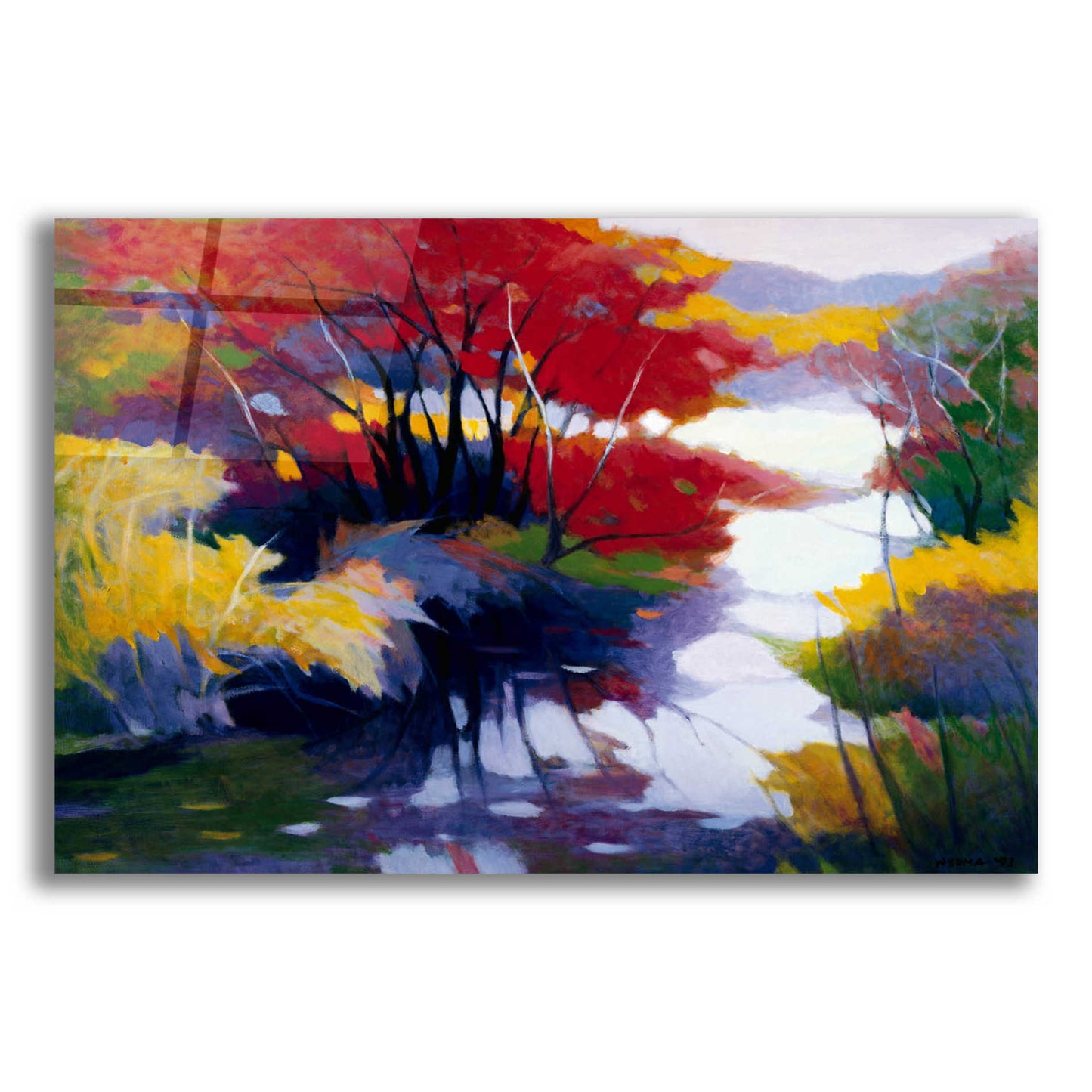The image appears to be a vivid painting, possibly created with watercolors given the subtly blended and occasionally running textures, although the colors seem more vibrant and dark than typical watercolors. The scene depicts a striking outdoor setting with a serene body of water, likely a lake or stream, which clearly reflects the surrounding flora. Dominating the foreground are brilliantly colorful flowers, featuring deep rust-red and gold hues, interspersed with flowers that have yellow petals, white fronds, and blue stems. To the right, similar flowers are present but less vibrant and fewer in number. The distant background features a hazy blue-gray sky partially obscured by shadowy mountains, contributing to the picturesque and tranquil atmosphere.